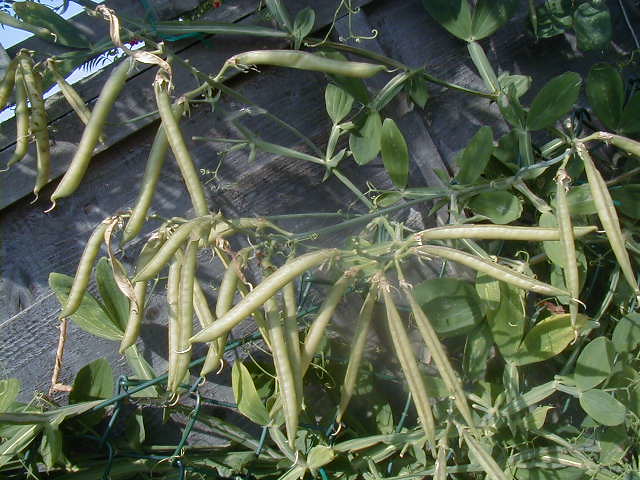This is a detailed close-up photograph of a flourishing green beans plant in an outdoor garden. The beans, light green and appearing ripe, hang prominently from the plant's long, curly vines. Approximately 25 to 30 beans can be seen, slightly out of focus at the center. The plant's leaves are a darker green, providing a contrasting background to the lighter beans. Also visible in the shot are unsuspecting small green flowers. Behind the plant, there's a dark, old, wooden wall, and a gray cement wall behind that. In the lower left corner, a green chain-link fence peeks into the frame. The upper left portion of the image captures a patch of blue sky with sunlight reflecting gently on the beans, suggesting a sunny day.